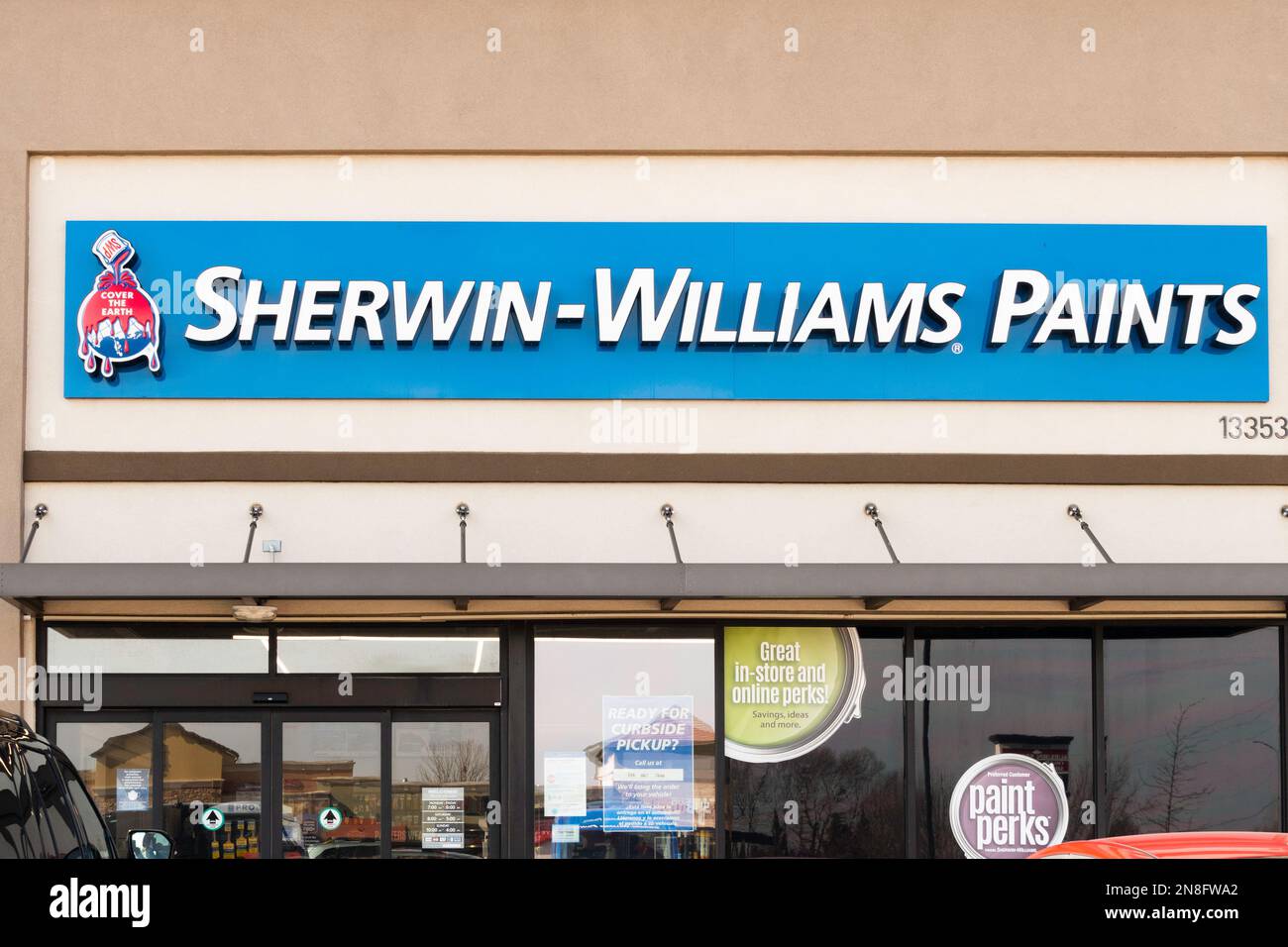The image depicts a modern Sherwin-Williams paint store, featuring a welcoming aesthetic with a tan awning and floor-to-ceiling windows. The store's sign prominently displays "Sherwin-Williams Paints" in white font against a dark blue background, accompanied by the company's iconic logo in the upper left corner. This logo showcases a red paint can spilling paint over a globe, symbolizing the company's slogan "Cover the Earth," which is faintly visible behind the main text in a subtle light blue.

In front of the store, a red car is partially visible, adding a pop of color to the scene. Notable signage includes a banner advertising "Paint Perks" and another sign promoting great in-store and online perks, encouraging customers to pick up their paint with ease. Upon closer inspection, the store's windows reflect surrounding buildings, adding depth to the image.

In the lower right corner, the image credits "ALMY" and provides the website "www.almy.com", suggesting that the content is brought to you by this entity. The overall impression is of a clean, inviting retail space designed to attract and serve customers effectively.